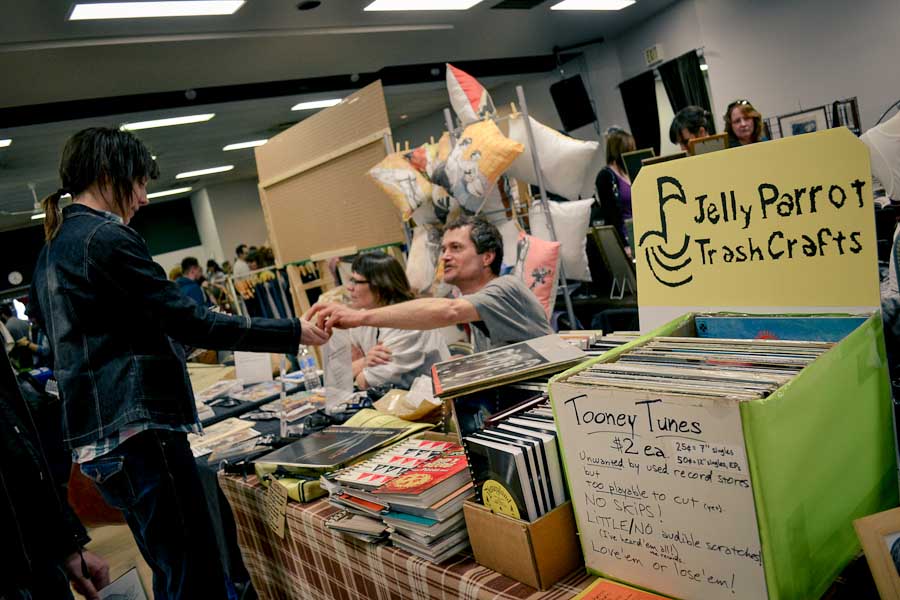In this bustling store, a table in the foreground is layered with an assortment of items, possibly including books, notebooks, and music records. Two individuals are seated at the table, with one person extending their hand across it. In front of the table, a woman stands wearing a matching jean jacket and jeans, her hand similarly outstretched, likely receiving change for a recent purchase. The background features a vibrant display of pillows hanging on the wall. Surrounding the scene, several more customers browse the store. Dominating the foreground is a large, green-covered box, prominently labeled "Jelly Parrot Trash Crafts" at the top. Written on the front of the box, against a white background, the text reads "Toonie Toons, $2 each." The scene encapsulates the lively atmosphere and eclectic offerings of this unique shop.